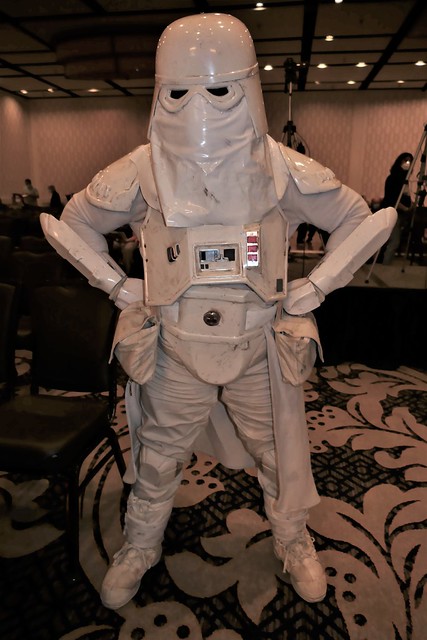At a bustling convention, an individual is captured in full gear resembling a stormtrooper from the Star Wars franchise, albeit with some notable differences. The figure stands confidently with hands on their hips, amidst a banquet room in a hotel, easily identifiable by the patterned carpet featuring a large blue and white floral motif. The armor, though evidently crafted for cosplay, is quite distinctive; it includes a heavy-looking, white head-to-toe ensemble with simple white pants and running shoes. The cosplay helmet, complete with a drooping plastic piece below the goggles, covers the head entirely, concealing the person's neck and adding a unique twist to the usual stormtrooper look. In the background, a few casually dressed convention-goers can be seen, contrasting sharply with the detailed and somewhat makeshift stormtrooper costume. The room's ceiling is dotted with lights and has a mix of dark and white panels, adding to the convention ambiance.